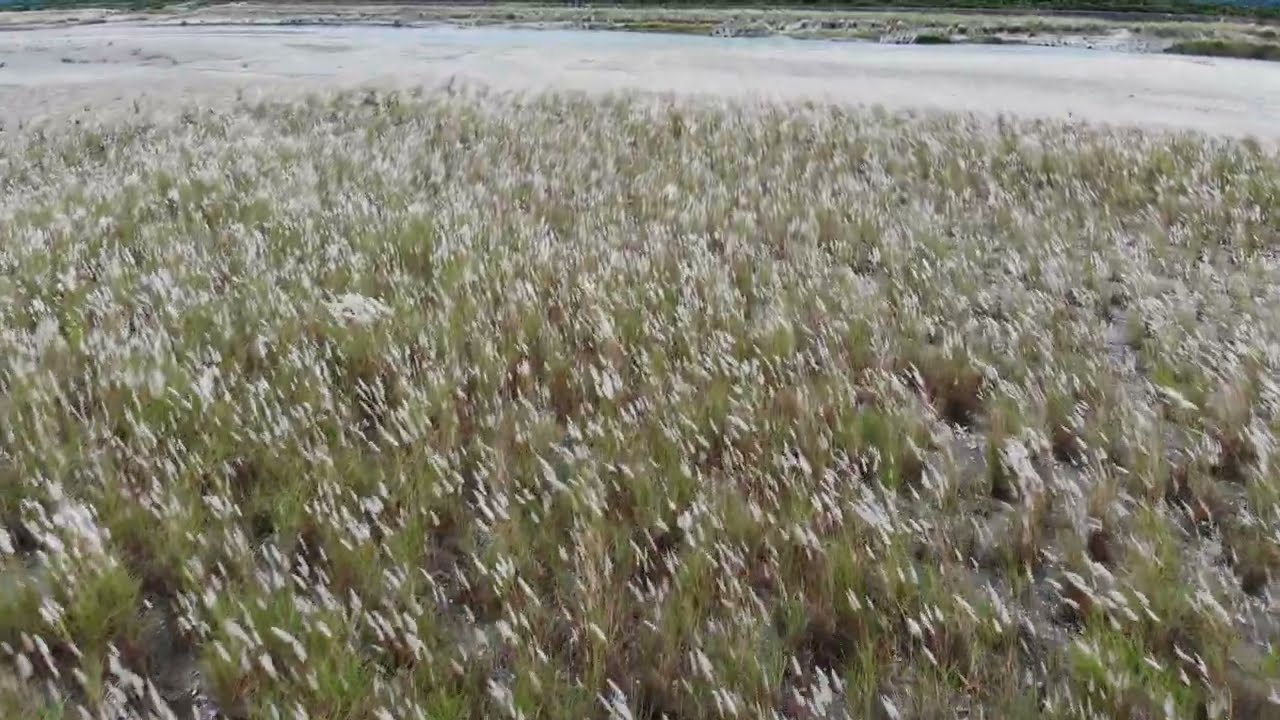The image is an outdoor photograph taken from a low angle, roughly knee-height, and features a large field dominated by tall grass with some white flowery tips, possibly milkweed or similar plants. The foreground grasses and weeds appear blurred, likely due to wind motion, giving a sense of movement across the frame. The lower 80% of the image highlights this dense green field, while the top 20% reveals a strip of barren hillside composed of sandy or coarse dirt. This sandy strip stretches horizontally from the left edge to the right edge of the image. Just beyond the grassy expanse, where the coarse dirt transitions into finer sand, there's what appears to be an inlet of water bordered by the raised, sandy terrain, creating a subtle shoreline effect. The lack of visible light source or shadows suggests an evenly diffused lighting, typical of overcast conditions.